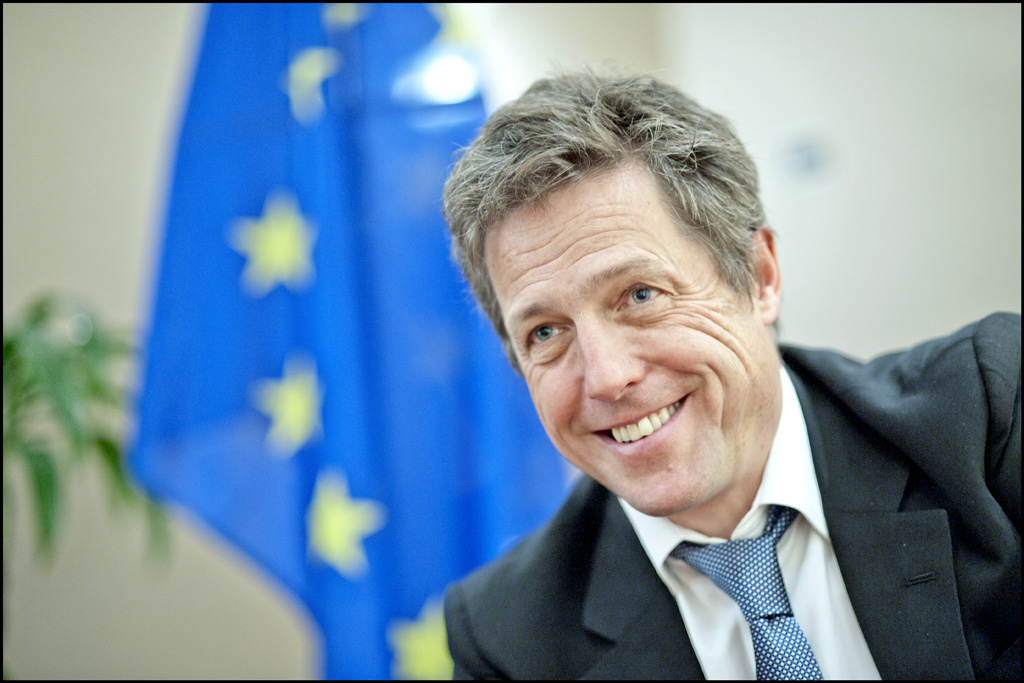This photograph features British actor Hugh Grant, who is prominently positioned on the right side of the frame, leaning slightly towards the center with a genuine smile on his face. His salt and pepper hair and visible wrinkles suggest this is a more recent picture of him. He is sharply dressed in a dark gray, slightly crumpled suit, paired with a white button-down shirt that is unbuttoned at the collar. His tie is a blue shade adorned with small white polka dots. Behind him, the background is out of focus, but you can make out a neutral white wall, a green plant on the left, and a blue flag featuring yellow stars towards the middle of the image. The flag and the setting suggest an official or governmental indoor space, though Hugh Grant himself does not appear to be posing formally, lending a candid feel to the photograph.